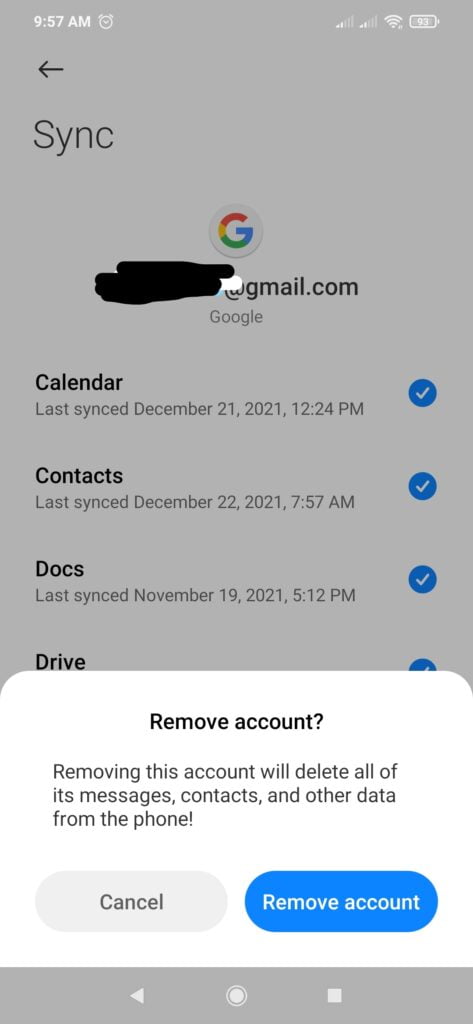In this image, we see a smartphone screen with a gray background. At the bottom of the screen, there is an open white dialogue box with the message: "Remove account?" Following the question, it states, "Removing this account will delete all messages, contacts, and other data from the phone." Below this message, there are two options: a gray "Cancel" button and a red "Remove account" button.

Beneath this dialogue box, the phone’s navigation keys are visible: a triangle icon for 'go back,' a circle icon for the home screen, and a square icon for multitasking.

At the top-left corner of the screen, the time is displayed as "9:57 AM" alongside a clock emoji. On the top-right corner, there are status icons indicating two bars of cell phone signal strength, a Wi-Fi signal, and a battery icon.

Underneath the top bar on the left side, a back arrow is visible. Below it, the word "Sync" appears, followed by the Google logo in the center of the screen. Next to the logo is a blurred-out email address where the first half is blacked out.

Further down, the word "Google" appears, followed by several lines of text detailing synchronization statuses: "Calendar - Last synced: December 21, 2021, 12:24 PM," "Contacts," "Docs," and "Drive." To the right of each of these items, there’s a blue circle icon containing a white check mark, indicating successful synchronization.